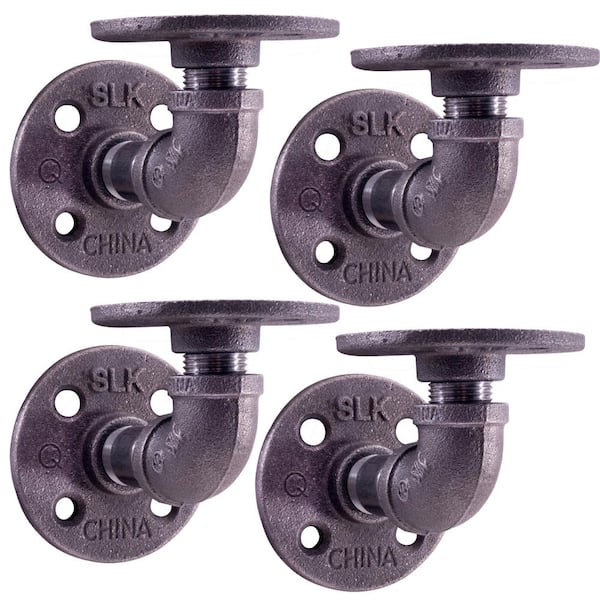This image depicts four identical pieces of sturdy gray metal equipment, arranged in a grid with two pieces in the top row and two in the bottom row, against a pure white background. Each piece features a round metallic base with four mounting holes, one at each edge forming a square pattern. Engraved letters "SLK" appear between the top two holes, while "China" is engraved between the bottom two holes. Extending from the center of each base is a short, curved cylindrical segment reminiscent of a plumbing pipe, although it does not seem intended for water use. Surmounting this curved pipe is a ridged metal component, which leads to a small circular flat platform at the top. The overall construction suggests a possible use for holding or displaying items, such as a candle or book. The equipment has a uniformly dirty metallic finish.